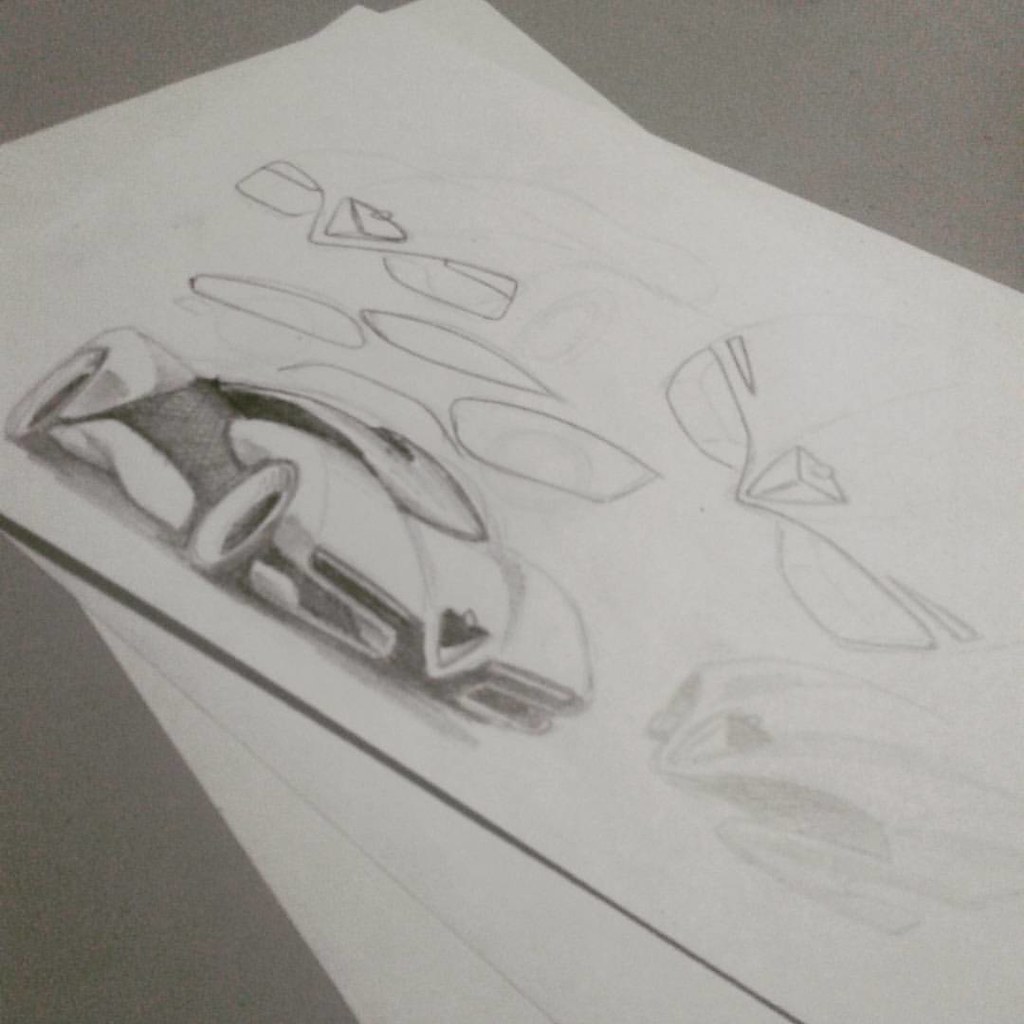A detailed pencil drawing of a sports car is showcased on a piece of white sketch paper, which rests atop several other white sheets on a gray surface, likely a table or countertop. The sports car bears resemblance to a Corvette, characterized by its sleek and curved hood. Prominently displayed in the middle of the hood is an emblem shaped like an inverted triangle, rendered in white and a darker color.

The vehicle appears to be white, accentuated by a dark stripe running along the side, starting from the front wheel and extending to the back. This stylish car design features a very low ground clearance, emphasizing its sporty aesthetic. The large wheels are complemented by whitewashed tires, further enhancing the automobile's sleek look. The low hood design suggests that the seating position inside the car is very low, offering a driver an intimate connection with the road while seated in the front seat.